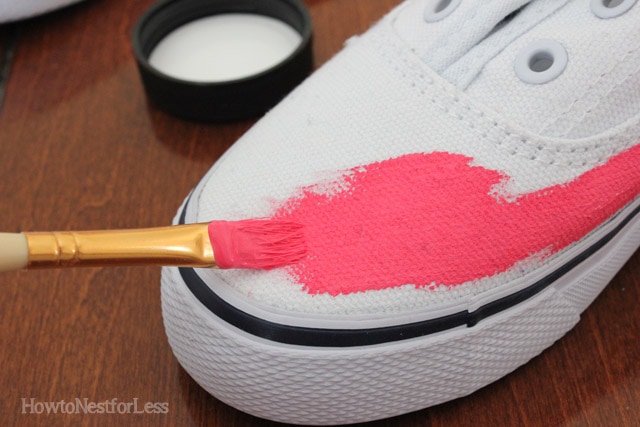The image features a close-up view of a white canvas shoe that resembles a classic Vans style. The shoe is positioned diagonally, extending from the center to the top right corner of the frame and lacks laces. The tip and left side of the shoe are partially covered in vibrant pink paint, applied using a paintbrush. The brush, adorned with a gold metal band above its bristles, is situated towards the bottom left of the image with its tip covered in the same pink paint. The shoe rests on a dark brown, wooden platform, adding texture to the scene. In the background, there is an out-of-focus black cup with a white interior. Additionally, there is slightly transparent white text in the lower left corner that reads, "How to nest for less." The overall composition captures the moment of artistic transformation with detailed elements of texture and color contrast.